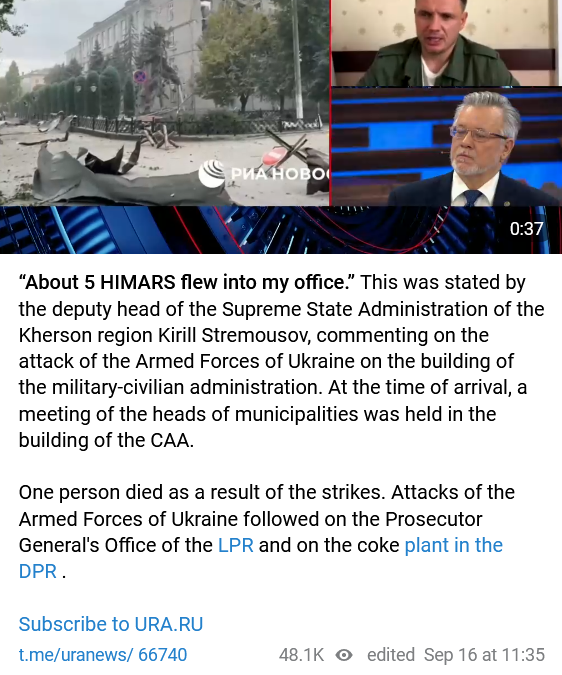The image is divided into three sections. The top part contains three photos: one on the left and two on the right. The left photo depicts a war-torn area, while the two on the right feature different men. A section below displays a timestamp reading "0:37." Below this, there is a caption that reads:

"About five HIMARS flew into my office."

- This statement was made by Kirill Stremousov, Deputy Head of the Supreme State Administration of the Kherson Region, in response to the attack by Ukrainian armed forces on the Military Civilian Administration building. During the strike, a meeting of the municipality heads was taking place inside the building, resulting in one fatality. Additionally, the Ukrainian armed forces carried out assaults on the Prosecutor General's Office of the LPR and the Koch plant in the DPR. 

- Subscribe to URA.ru and follow at T.ME/URANEWS/66740.